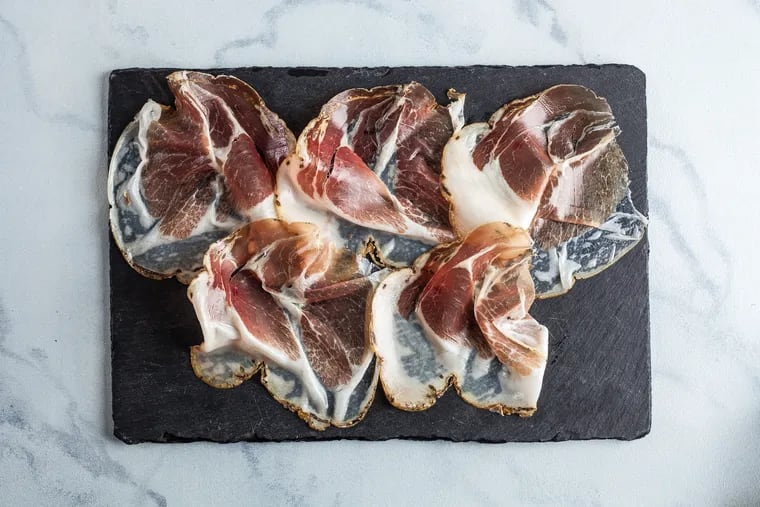The image features a top-down view of a rustic scene centered on a marbled countertop. Atop this marbled surface lies a natural-looking, black stone cutting board, which appears chiseled with imperfect edges. Displayed on this cutting board are five thinly sliced, uncooked pieces of meat. The meat has a rich reddish-brown color marbled with white fat, suggesting it could be prosciutto or a similar type of cured ham. The slices are arranged in two overlapping rows, with three pieces on the top row and two on the bottom. Some slices appear slightly translucent, revealing parts of the cutting board beneath. Additionally, there is a subtle seasoning blend visible along the edges of the meat, enhancing its artisanal appearance.